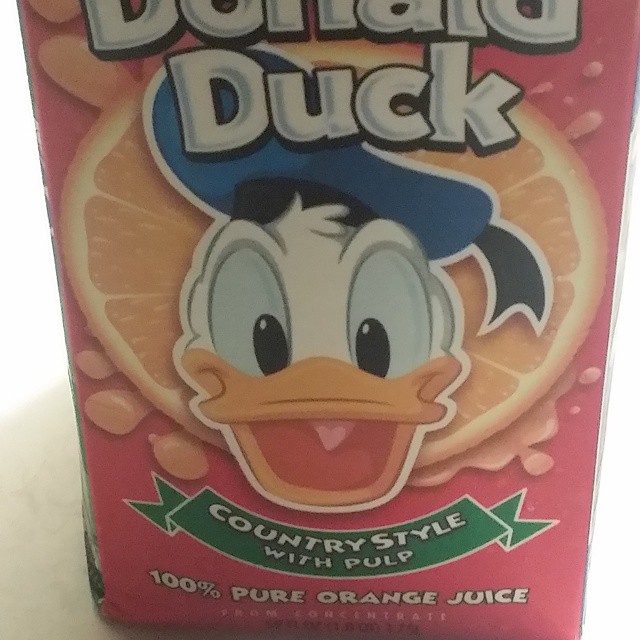The image is a close-up photo of a Donald Duck orange juice carton. The top portion of the carton is cropped out, emphasizing the central design elements. The carton features a prominent dark orange background with an orange slice at the center, overlaid by a forward-facing, happy and excited Donald Duck. His blue hat, white face, light blue eyes with black pupils, and orange beak are accentuated against the orange slice backdrop. Surrounding the orange slice are illustrated droplets of orange juice. Above Donald Duck’s face, "Donald Duck" is written in large white letters. Below this central image, a green banner outlined in white with pointed ends displays the words "COUNTRY STYLE WITH PULP" in capital white letters. At the very bottom of the carton, the text "100% PURE ORANGE JUICE" appears, followed by "FROM CONCENTRATE," both in white lettering. The background beneath the carton is white, with a slight gray shading in the bottom left corner, although the main focus remains entirely on the juice carton.